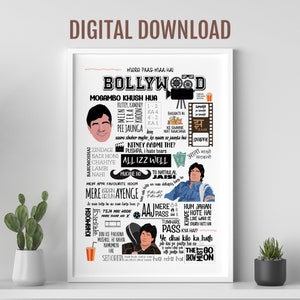This square image features a gray background with a white rectangular centerpiece. At the top of the gray background, the text "DIGITAL DOWNLOAD" is prominently displayed in brown, uppercase letters. Flanking the central white rectangle are two potted plants: on the left, a taller cactus in a white ceramic pot, and on the right, a smaller succulent in a gray pot.

Within the white rectangular frame, the word "Bollywood" stands out, using two of the O's to form part of a black video camera illustration. Below "Bollywood" on the left side, there's an image of a man's face with dark hair, and beneath the video camera on the right, there's a film reel graphic. Further down, there's a depiction of a man in a blue shirt, showing his torso and face, followed by another man dressed in dark colors in the center. A red drink cup is situated in the bottom left corner of the white rectangle. The content inside the white rectangle is dense with text, though most of it is too small to read clearly. The overall composition resembles a collage, blending elements of Bollywood-themed imagery, such as caricatures or drawings of actors, and various graphics like a mustache and a film strip.